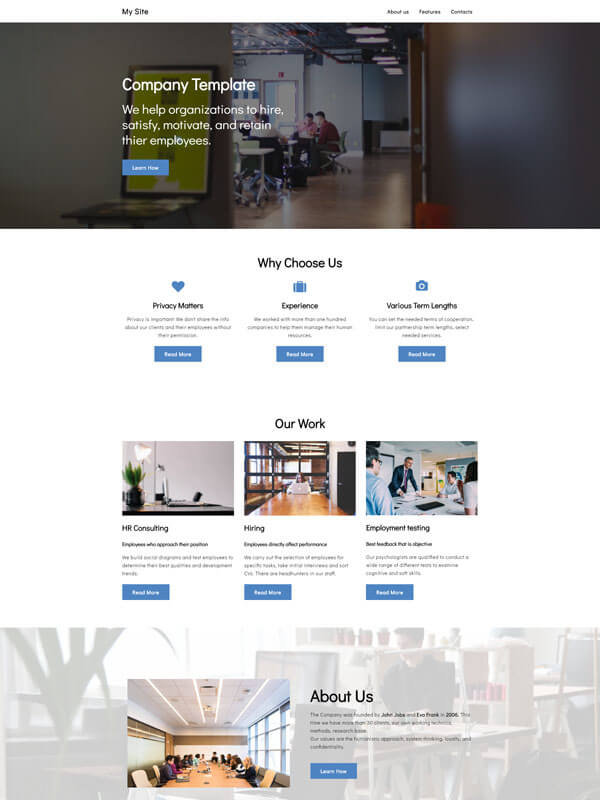In the top left corner, written in black text against a white background, is the title "MySite". On the top right, smaller text displays the menu options: "About Us", "Features", and "Contacts". Below, there is a large office setting featuring grayish-black walls, wooden floors, and several desks where people are seated. Prominently displayed in white text is the header, "Company Template". The text caption reads, "We help organizations to hire, satisfy, motivate, and retain their employees." Below this, a blue box with white font contains the call-to-action "Learn More".

Centered beneath the main header, bold black text asks, "Why Choose Us?" followed by icons: a heart, a briefcase, and a camera, each in blue, representing Privacy Managers, Experience, and Various Term Links respectively. Accompanying gray text, which is difficult to read, presumably offers further details. Underneath, three blue boxes, each labeled "Read More" in white text, provide additional information.

Further down, black text introduces the section titled "Our Work", accompanied by generic stock photos. These images relate to HR consulting, hiring, and employment testing, supplemented by extensive, unreadable text. Each section includes the same blue boxes with white callouts. 

At the bottom of the page, another typical boardroom scene appears to the right, labelled "About Us", followed by a blue information box similar to the previous ones. This section wraps up the content displayed in the image.